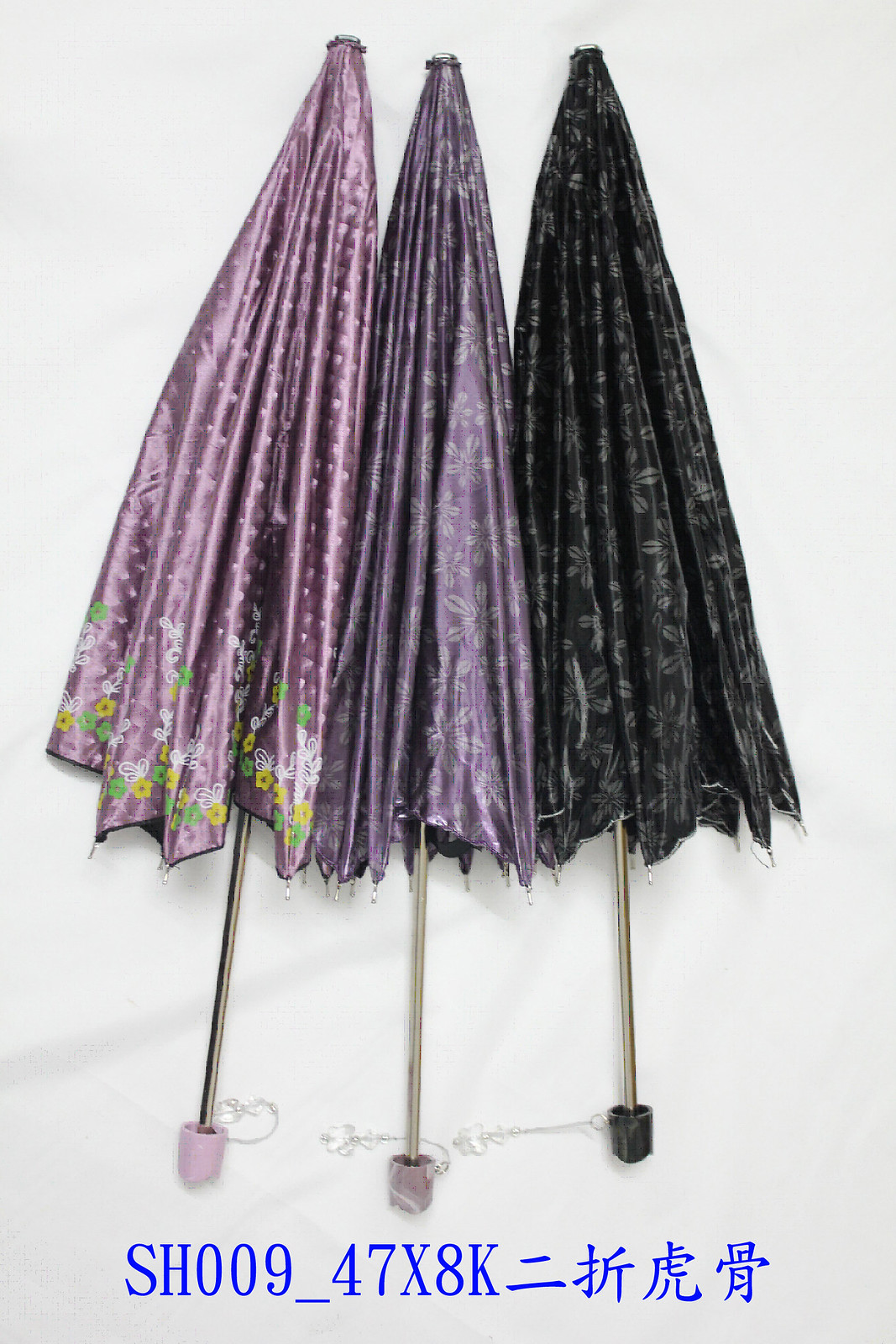This product photograph showcases three vertically standing, closed umbrellas with extended handles, set against a white background. Each umbrella boasts a distinct, shiny fabric and is adorned with unique patterns. From left to right, the first umbrella is a lighter purple, embellished with intricate floral designs in white, green, and yellow near the bottom. The central umbrella features a deeper purple hue with white floral patterns. The umbrella on the right is black and decorated with subtle gray floral motifs alongside what appears to be gold lettering. Each umbrella is equipped with a small handle at the bottom, from which tiny charms dangle - although the exact shapes of these charms are indistinguishable. Below the umbrellas, in blue text, is the alphanumeric code "SH009-47X8K" followed by what seem to be Japanese or Chinese characters.